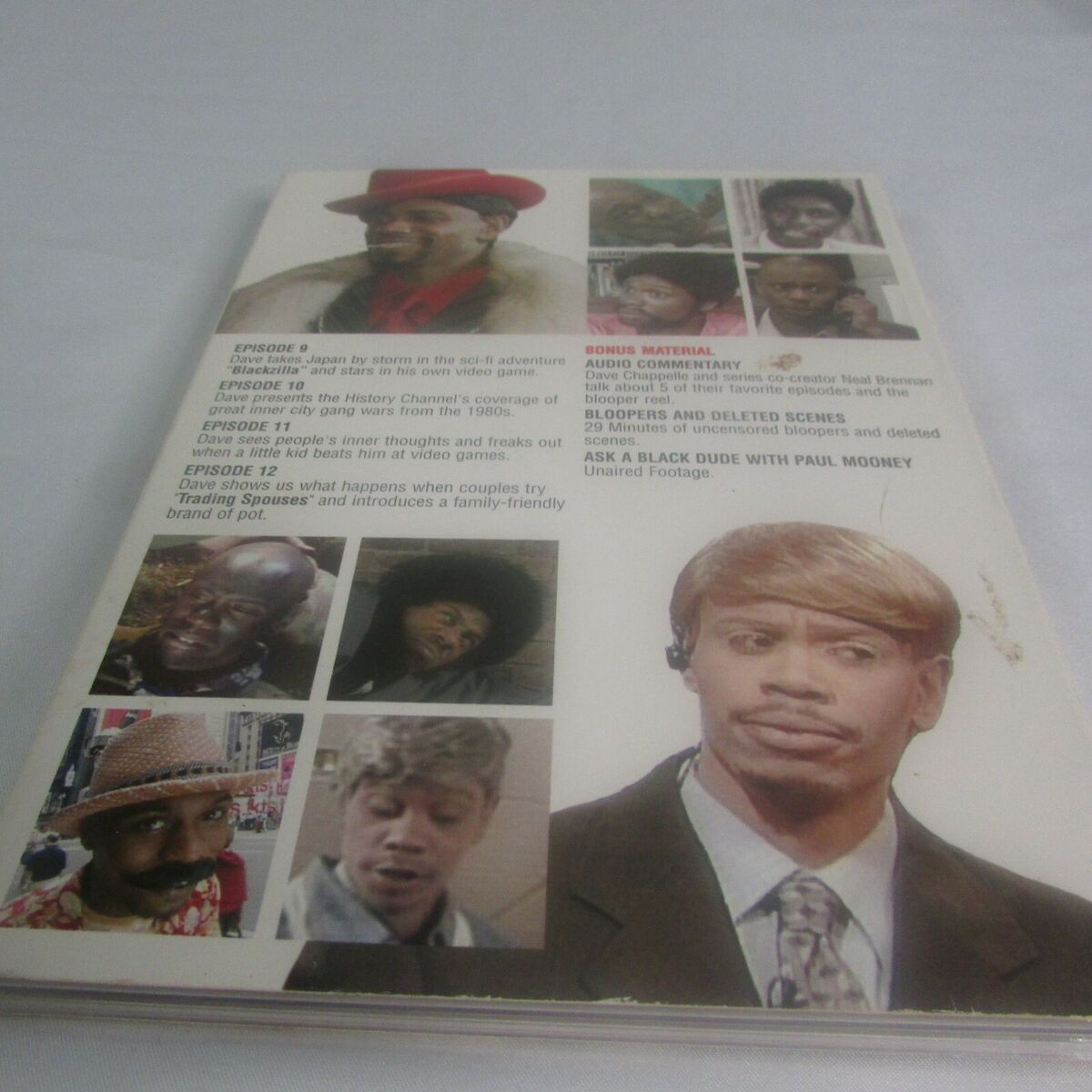This is a square, somewhat blurry image of a worn hardcover book cover, set against a light gray background, possibly a counter or table. The cover is predominantly white, marred by brown stains at the top and bottom on the right side. It prominently features numerous images and text.

In the upper left corner, a square section showcases an African-American man wearing a red hat, a red bowtie, and a fuzzy white coat over his shoulders. To the right of this image, four smaller pictures of African-American actors are displayed. Similarly, in the lower left corner, there are four more smaller pictures of African-American actors. The lower right corner is dominated by a larger image of an African-American actor with a light brown wig, dressed in a suit and tie. 

In the center, the headings indicate an episode guide with the text: "Episode 9" followed by two lines of descriptive text, "Episode 10" with two lines of text, "Episode 11" with two lines of text, and "Episode 12" with three lines of text. To the right, in red, the text reads "Bonus materials," listing "audio commentary," "bloopers," and "deleted scenes."

Additionally, the content and characters are tied to Dave Chappelle's "Chappelle's Show," featuring various characters from the show, including recognizable figures like Rick James and the black KKK guy, among others. The text also features the phrase "Ask a Black Dude with Paul Mooney," indicating a segment from the show.